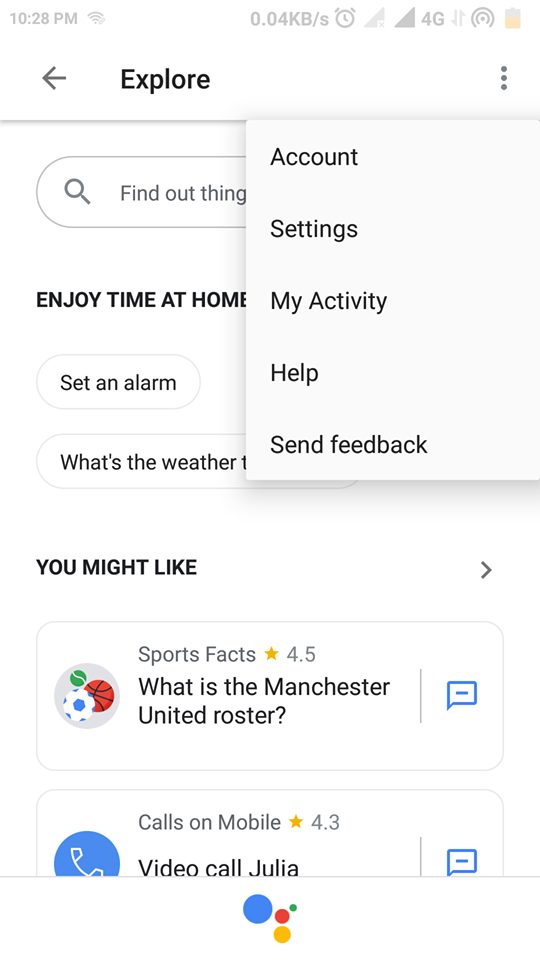The image is a screenshot of a mobile phone screen with a primarily black text on a white background. 

At the top of the screen, displayed in grey text, is the time, "10:28 PM," positioned on the left-hand side. Adjacent to the time is a series of status icons: a Wi-Fi icon, a clock icon showing a data transfer rate of "0.04 kbs per second," two 4G signal indicators (one fully filled), a possible mobile hotspot icon, and a half-full battery icon.

Below this status bar, in black text, is the word "Explore," flanked by a back arrow to the left and a hamburger menu on the right. The hamburger menu is expanded, revealing options such as Accounts, Settings, My Activity, Help, and Send Feedback.

Moving down, on the left-hand side, part of a curved search box is visible with the prompt "Find out things" inside it. Underneath the search box, a series of suggestions are listed: "Enjoy time at home," "Set an alarm," and "What's the weather."

Further down, there is a section titled "You might like," accompanied by a forward arrow. Within this section, there are two rectangular items:

1. The first rectangle is a sports-related card titled "Sports Facts" with a 4.5-star rating. It poses the question, "What is the Manchester United roster?" To the left, there is a grey circle featuring three footballs in red, white, blue, and green. A blue message icon is placed to the right of this card.

2. The second rectangle is titled "Calls on Mobile," with a 4.3-star rating, featuring a video labeled "Julia." It has a blue circle with a white phone icon on the left side and a blue message icon to the right. Part of the text and bottom of the icon seems to be cut off.

At the bottom center of the screen, a few colored circles are visible: a blue one to the left, a smaller red one next to it, a tiny black circle, and below the red one, a small yellow circle.